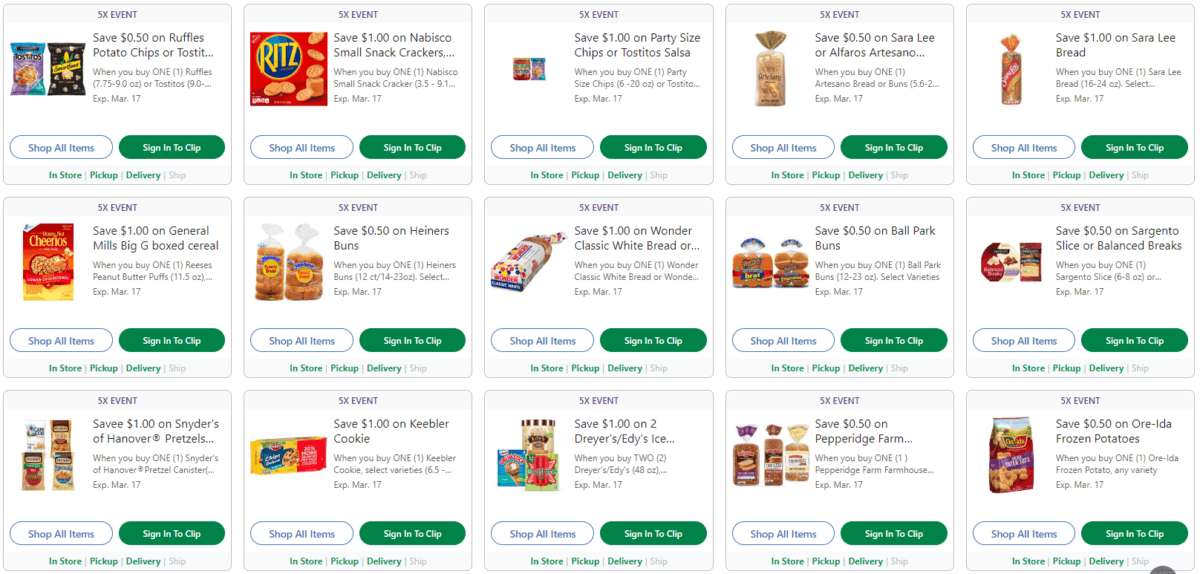Screenshot of a coupon-based website displaying various grocery items, arranged in a grid with 5 columns and 3 rows. Each product card lists potential savings and features two buttons: a "Sign in to Klip" button on the right, and a "Shop All Items" button on the left. The top of each product card prominently displays "5x Event." 

The first column, from top to bottom, shows:
1. A bag of chips 
2. Another bag of chips 
3. Cheerios cereal.

The second column includes:
1. A box of crackers 
2. A loaf of bread 
3. Hamburger buns.

The third column features:
1. Another loaf of bread 
2. More hamburger buns 
3. Cheese slices.

The fourth column displays:
1. What appears to be a pretzel bag 
2. Different types of cookies 
3. Various ice cream products.

The fifth column consists of:
1. Another loaf of bread 
2. What looks like frozen french fries or potatoes 
3. Another type of bread.